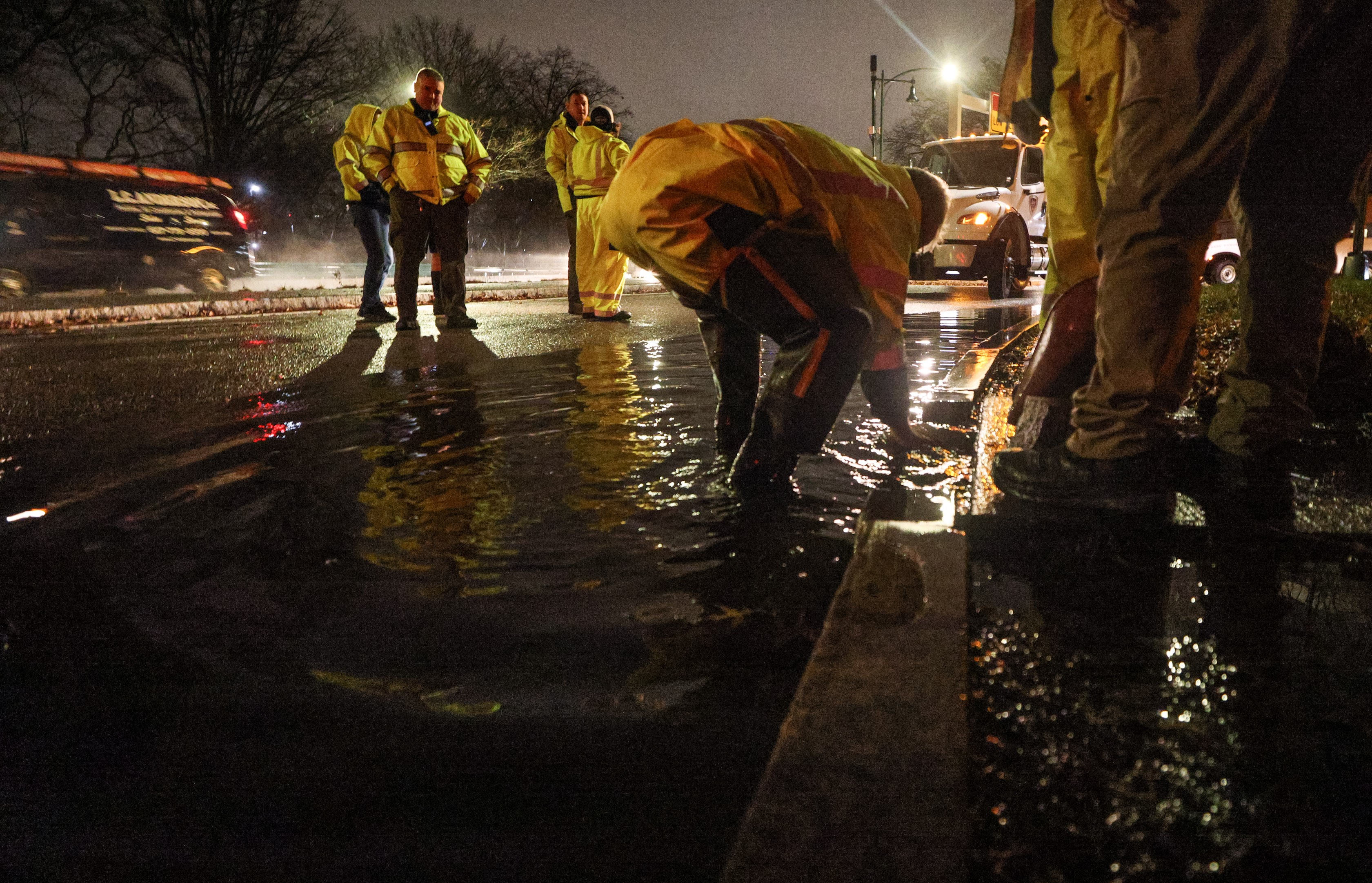This is a night-time photograph captured during a storm or flood, with a distinctly urgent atmosphere. It shows a team of municipal workers dressed in reflective yellow rain gear, wading through large puddles caused by an apparent drain blockage. The scene is illuminated by streetlights and work truck lights, casting a mix of yellows, dark browns, and blacks across the image. Central to the photo is one worker bending down, hand in the water, likely attempting to unclog a drain at the curbside. Behind him, other workers are either observing or conversing. In the background, various vehicles including a white rescue truck and a dark-colored work truck with white writing are visible. The camera angle is low, almost as if placed on the sidewalk, emphasizing the severity of the flooding issue being addressed.